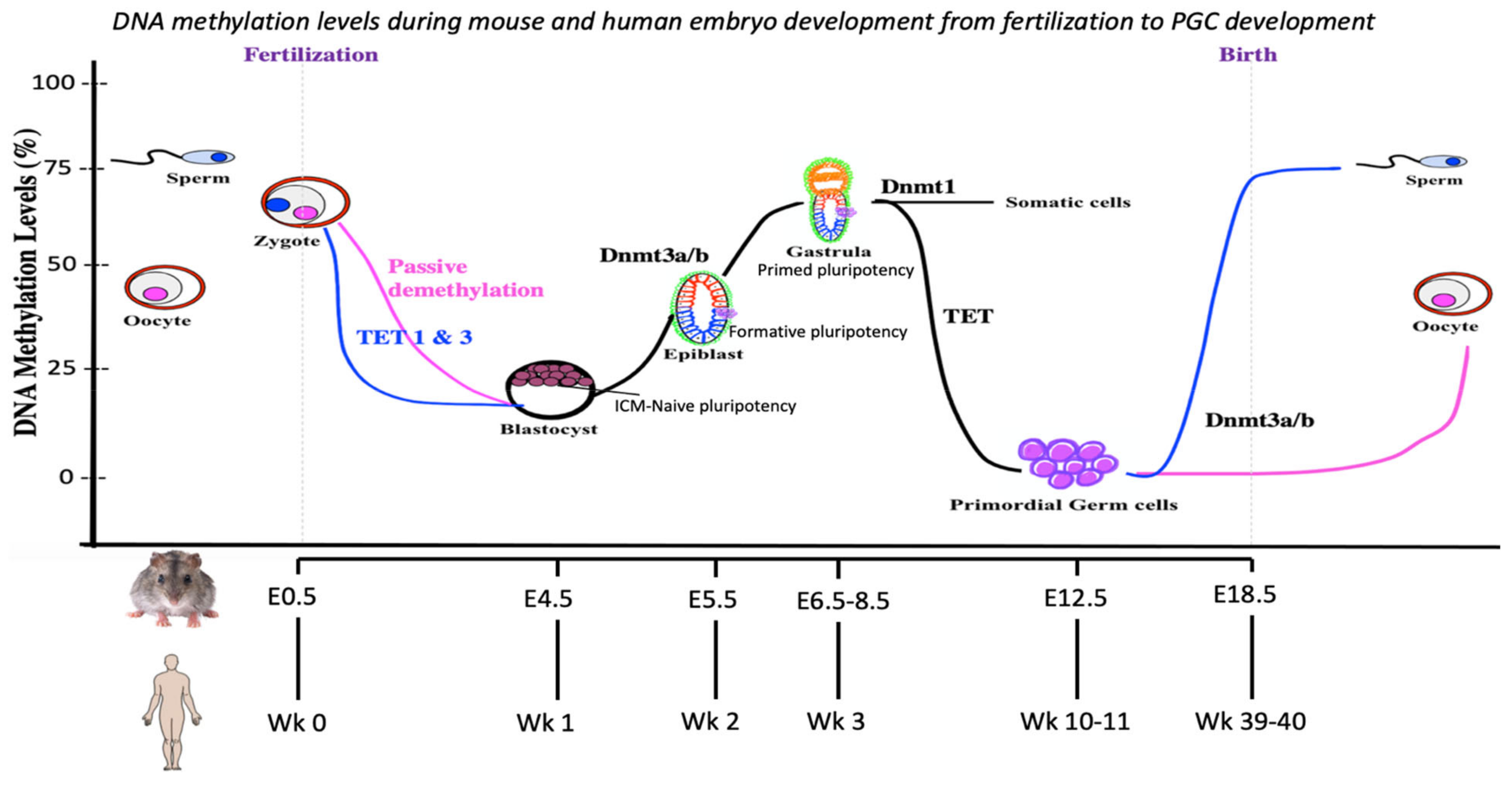The image is a detailed chart depicting DNA methylation levels during mouse and human embryonic development from fertilization to the development of primordial germ cells (PGCs). The title at the top reads "DNA Methylation Levels During Mouse and Human Embryo Development from Fertilization to PGC Development." The y-axis on the left is labeled "DNA Methylation Levels Percent" and ranges from 0% to 100% in increments of 25%. The x-axis at the bottom provides a timeline for both mouse and human development, marked as E0.5, E4.5, E5.5, E6.5 to E8.5, E12.5, and E18.5 for the mouse, and week 0, week 1 to week 3, week 10 to 11, and week 39 to 40 for the human.

Within the graph, various stages of development and demethylation are illustrated, starting from sperm and oocyte, moving through zygote formation, and detailing phases such as passive demethylation, TET1 and 3 involvement, blastocyst, inner cell mass (ICM), naïve pluripotency, epiblast (form of pluripotency), gastrulation, and primed pluripotency. Labels include DNMT1 somatic cells, TET, primordial germ cells, and DNMT3A/B, culminating in references to sperm and oocyte once again. The graph shows fluctuating methylation levels: the sperm's curve initiates and concludes at approximately 75%, while the oocyte's curve starts and ends around 50%, with both experiencing a sequence of descending, then ascending, and again descending trends. At the bottom center of the image, there are scaled illustrations of a mouse and a human to emphasize the corresponding developmental stages.